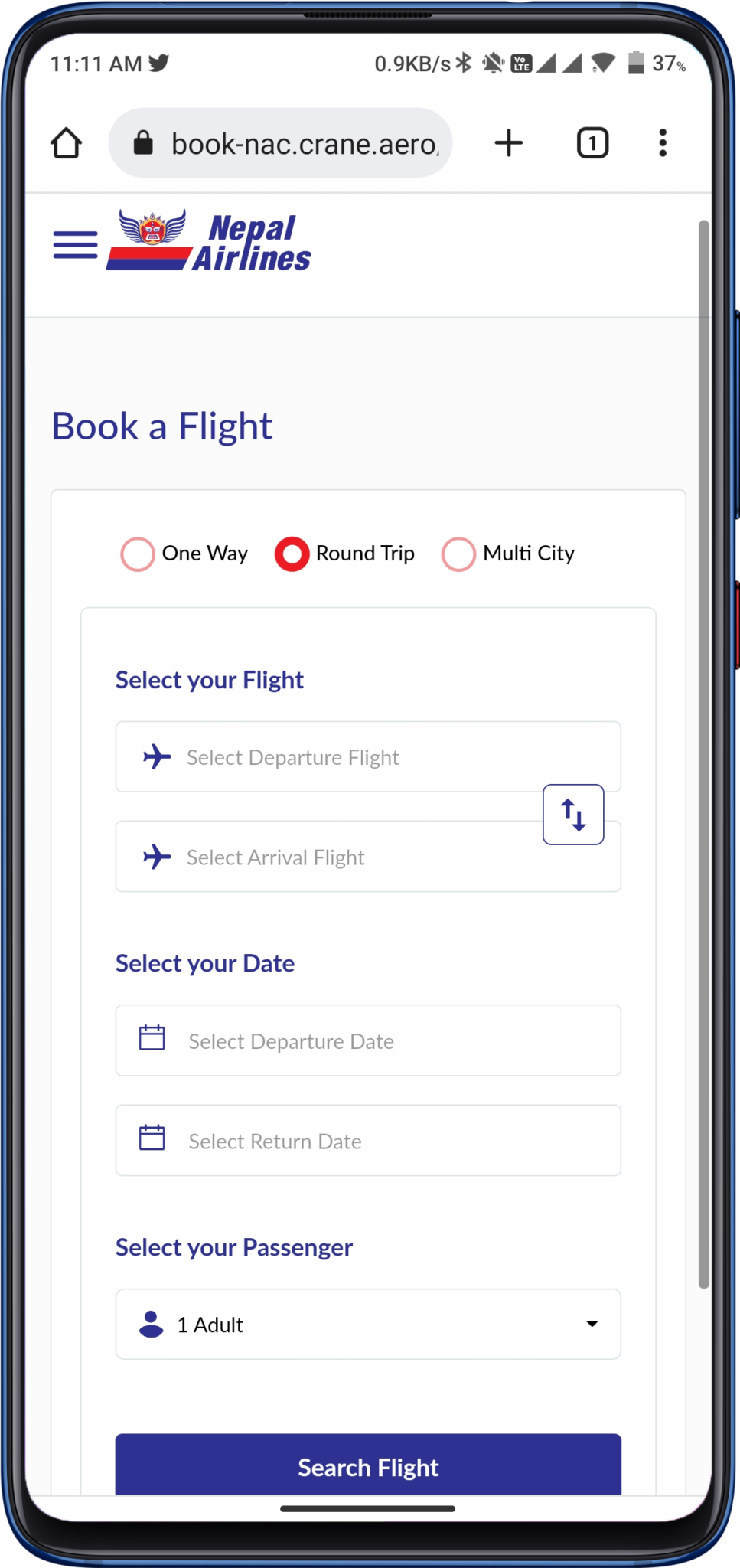A close-up image shows a blue smartphone displaying the Nepal Airlines website. The phone, which has two buttons on its right edge, indicates a 36% battery level, a Wi-Fi symbol, two cellular data symbols, an LTE icon, a no-notification icon, a Bluetooth symbol, and a data transfer rate of 0.9 kilobits per second at the top of the screen. The time reads 11:11 a.m. on the far left, alongside the Twitter logo.

The web browser in use appears to be Google Chrome, as evidenced by the home button, address bar (displaying book-nack.crane.aero), new tab button, tab button, and the three-dot settings menu. The webpage itself has a clean, white background with Nepal Airlines branding. In the top-left corner, a three-line icon indicates a drop-down menu, and next to it, the Nepal Airlines logo and brand name are prominently displayed. 

Below, options are available to book a flight, with the "Round-trip" option highlighted in red. Further down, sections for selecting flights, departure and arrival dates, and passenger numbers are visible. Specifically, the user can choose the departure and arrival flights, set the desired dates, and select the number of passengers (currently set to one adult). At the bottom, a large blue button prompts the user to "Search Flight."